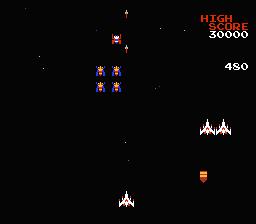This image is a screenshot from the classic video game, Asteroids. The background is entirely black, enhancing the retro aesthetic typical of early arcade games. In the upper right-hand corner, the high score is prominently displayed in red, reading "30,000," followed by the current score of "480." The screen features three white rocket ships, with one positioned at the bottom and two more along the right-hand side. At the center and towards the top of the screen, various objects and enemies are visible. These include other types of rocket ships in blue and red, as well as more abstract shapes that descend from the top. The central rocket ship is actively aiming at these targets, reminiscent of the dynamic gameplay typical of Asteroids.